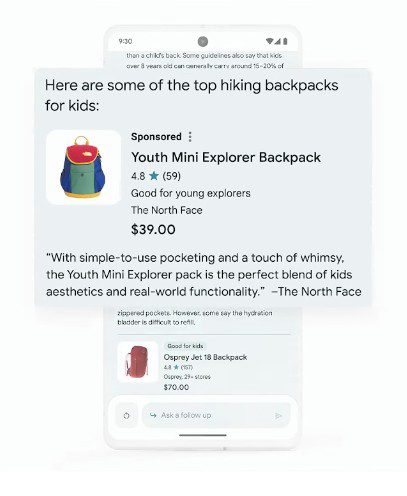The image showcases a mobile app interface designed for purchasing items, presenting a shopping experience on a white smartphone. The top-central area of the phone screen features a grayish-black camera symbol, with the current time displayed in the top left corner, and the Wi-Fi, battery, and cellular signal indicators in the top right.

A prominent black text is layered on the page, and a significant portion of the upper and central sections of the screen is dominated by a pop-up window. At the bottom section of the screen, there is an advertisement for a backpack, specifically the Osprey Jet 18 in red, which is marked as "Good for Kids." This product boasts an impressive rating of 4.8 stars based on 157 reviews and is priced at $70. An image of the red backpack appears to the left of these details.

Embedded in the pop-up, the app highlights "Some of the Top Hiking Backpacks for Kids." A picture of a colorful, multi-colored backpack is featured on the left side of the pop-up, accompanied by a "Sponsored" label. Below this, another product is detailed: the "Youth Mini Explorer Backpack," also rated 4.8 out of 5 stars from 59 reviews, priced at $39, and branded as "Good for Young Explorers" by The North Face.